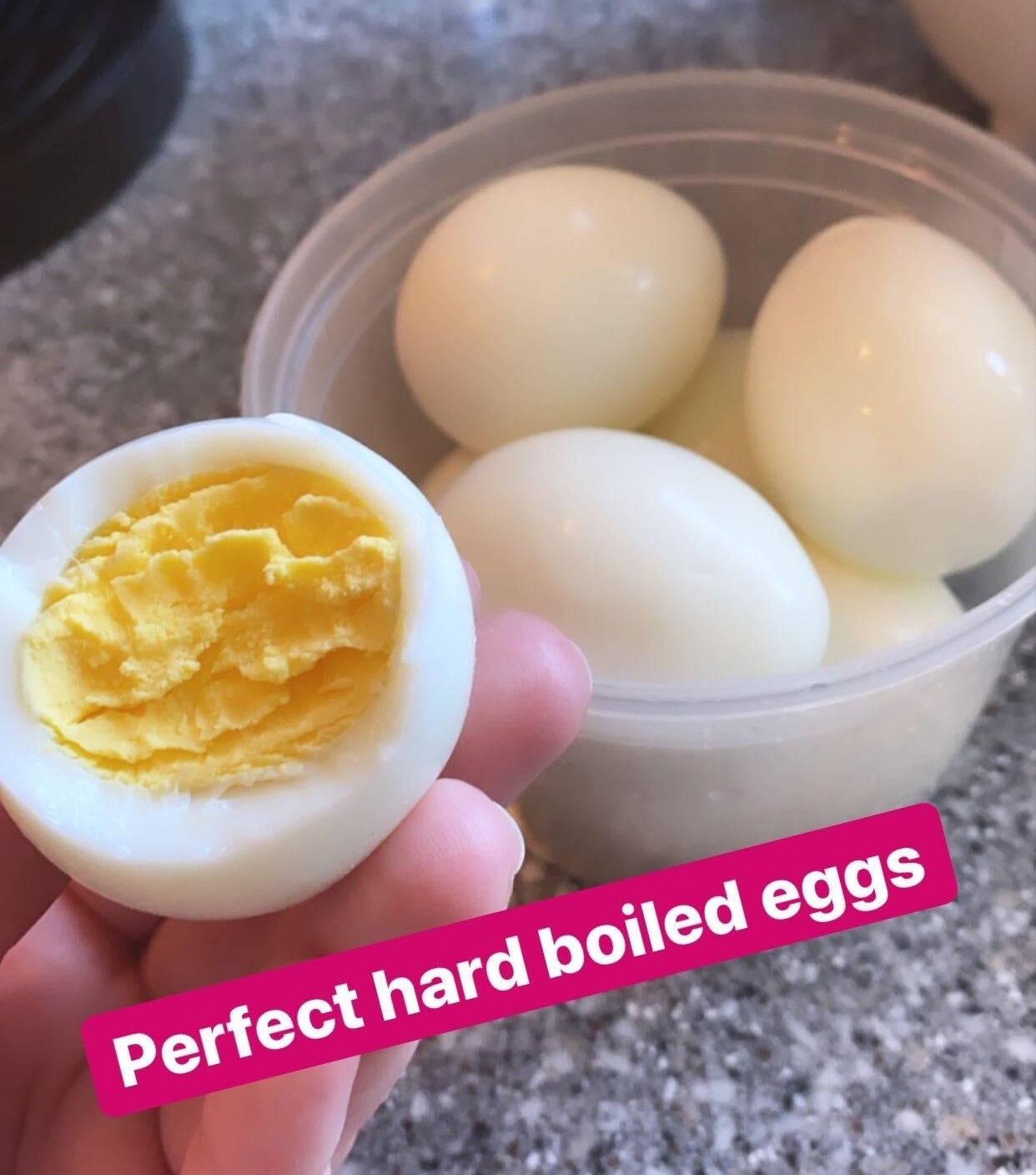In this image, which appears to be a still from a video, possibly from TikTok, there's a clear plastic container, shaped like a large cylindrical bowl, sitting on a polished, white and gray marble countertop. Within the container, there are approximately six hard-boiled eggs. To the left of the container, a woman's hand, with light skin, holds up a half-eaten hard-boiled egg, revealing a fully cooked, solid yellow yolk inside. Beneath the scene, the phrase "perfect hard-boiled eggs" is displayed in white lettering against a rounded pink rectangular border. In the background, though slightly obscured, there is black cookware in the top left corner and white cookware in the top right corner, adding to the kitchen setting.